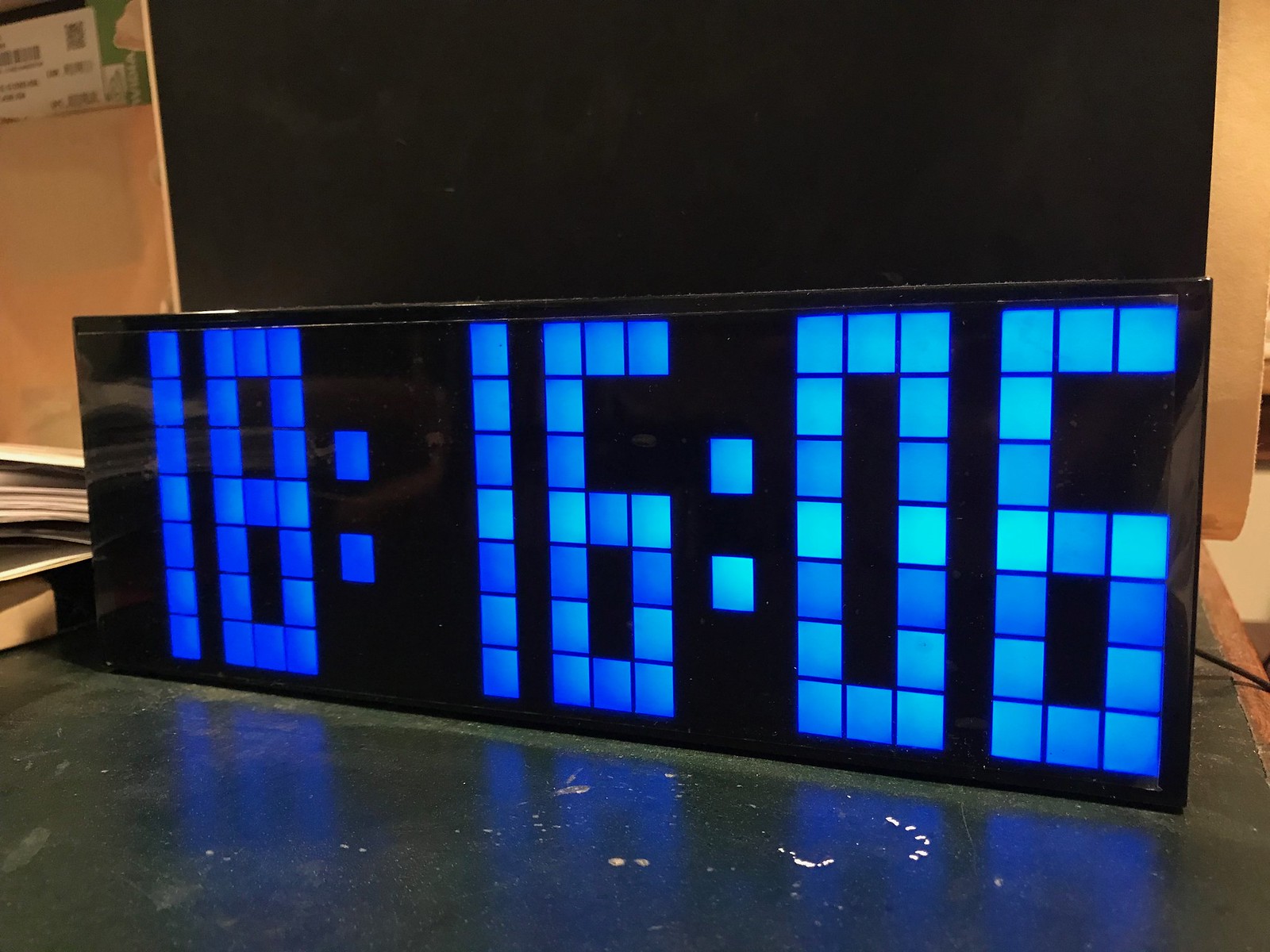The image captures a large rectangular black box displaying a digital countdown with numbers "18:16:06," presumably indicating 18 hours, 16 minutes, and 6 seconds. The display consists of blue LED squares forming the digits, with varying shades from dark to light blue. This box is placed on a desk with a green top, and to the left side, there are neatly stacked papers. The surroundings suggest a classroom or an office setting; there is a green-topped desk and a background that includes both a blackboard and bulletin board. Additionally, a brown wooden part of the wall and a contrasting light beige wall are visible, alongside a concrete floor marred with white scratches. Further in the background, a desk can be seen with a newspaper on it and possibly a small pink lamp. The setting gives off an organized yet busy atmosphere.